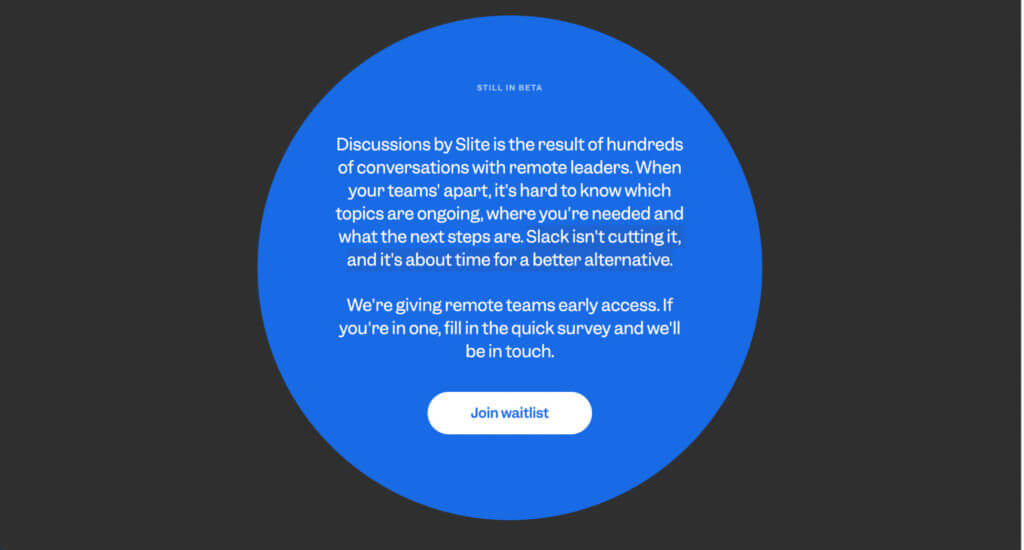A screenshot of a website features a central blue circle against a black background. Some white space appears on the right side, indicative of an incomplete screenshot. Within the blue circle, white text reads: "Discussions by slight is the result of hundreds of conversations with remote leaders. When your team is apart, it’s hard to know which topics are ongoing, where you're needed, and what the next steps are. Slack isn't cutting it, and it's about time for a better alternative. We're giving remote teams early access; if you're in one, fill in the quick survey and we'll be in touch." The top of the circle is labeled "Still in Beta." At the bottom, a white oval button labeled "Join Waitlist" invites users to click. The website appears to be an alternative communication tool for remote teams, akin to Slack, currently in the beta testing phase.